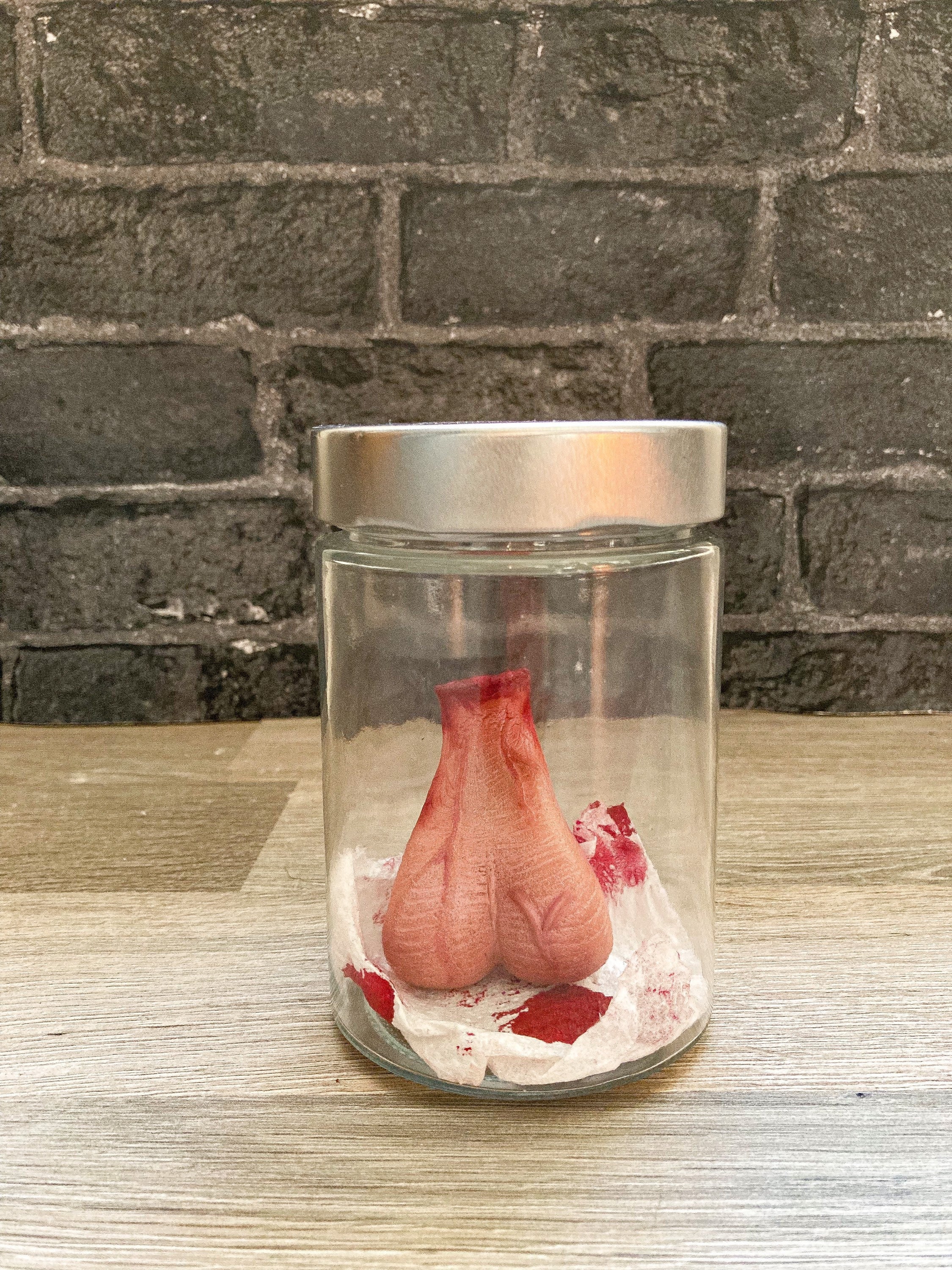In the image, a clear glass jar with a silver cap is prominently positioned on a grayish-beige wooden table. Inside the jar, there is what appears to be a human tissue resembling male testicles, placed on a napkin. The tissue, which is beige, is severed at the top, showing red and bloody details that suggest recent cutting. Dark splotches of blood are visible on the napkin beneath the tissue. The background features a dark gray brick wall, adding to the stark and somewhat eerie atmosphere of the scene. The clear visibility of the contents within the jar emphasizes the unsettling nature of the image.